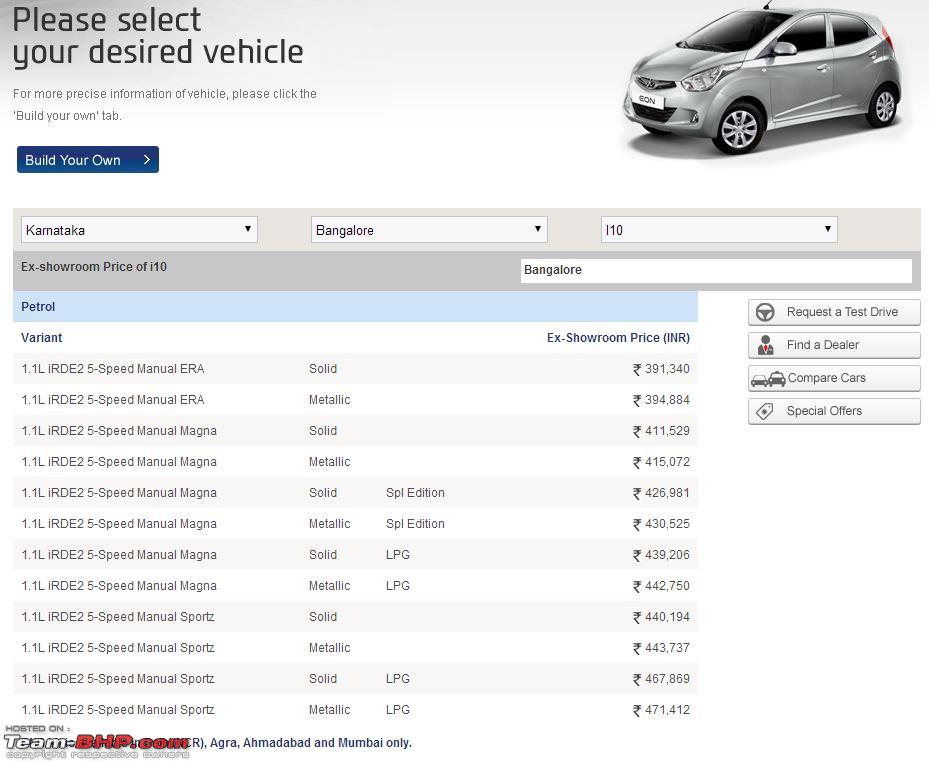The web page is designed to allow users to select and customize a Hyundai i10 vehicle based on their location and preferences. At the top of the page, clear instructions guide users on how to proceed, accompanied by a prominent "Build Your Own" button. Below these instructions are dropdown menus where users can select their state and city, specifically mentioning Bangalore, as well as the car model, which is the Hyundai i10.

The main section of the page provides detailed ex-showroom prices for various Hyundai i10 variants available in Bangalore, listed in Indian Rupees (INR) and categorized under petrol variants. Each variant entry includes descriptions of the engine specifications, transmission type, and paint options, which include solid and metallic finishes, as well as special edition options.

The available Hyundai i10 variants are:
1. 1.1L IRDE2 5-speed Manual
2. 1.1L IRDE2 5-speed Manual Magna
3. 1.1L IRDE2 5-speed Manual Magna LPG
4. 1.1L IRDE2 5-speed Manual Sport
5. 1.1L IRDE2 5-speed Manual Sport LPG
6. 1.1L IRDE 5-speed Manual Sport AT

On the right side of the page, there are buttons for additional actions, including "Request a Test Drive," "Find a Dealer," "Compare Cars," and "Special Offers." An image of a Hyundai i10 is prominently displayed at the top right corner of the page, enhancing the visual appeal and providing a preview of the vehicle.